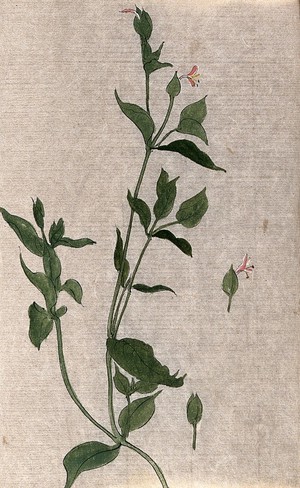The image depicts an old painting of a botanical subject, meticulously rendered on a piece of aged, tannish parchment or canvas paper. The texture of the substrate is evident, showcasing its fibrous or grainy quality, hinting that it has weathered the passage of time. Dominating the composition is a tall, green plant with elongated stems that ascend both vertically and to the left. The main vertical stem is accompanied by a few smaller tributary stems. The green leaves are pointed at the tips, featuring prominent central veins and smaller veins that segment the leaves into distinct sections.

Near the top of the plant, a delicate pink flower blooms, complete with stamens that boast yellow centers and black tips. Midway down the piece, a detached element—a leaf paired with another pink flower—adds an intriguing detail to the artwork. Additional detached leaves, seemingly pointing upwards, are positioned to the side, further complementing the botanical theme. The overall simplicity of the drawing, combined with the timeworn look of the parchment, imbues the image with a sense of historical artistry and delicate beauty.